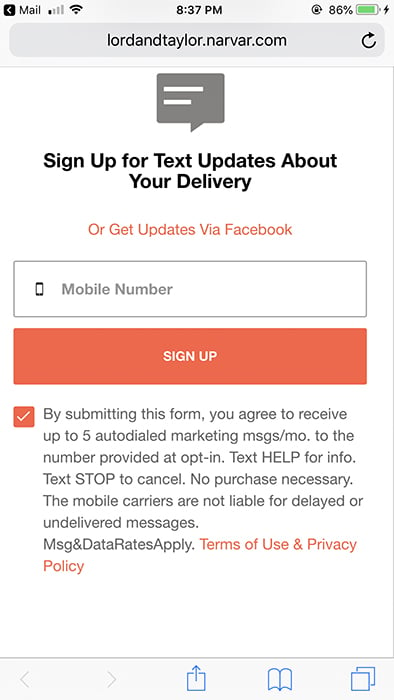This screenshot depicts a sign-up section on the Lord and Taylor website, hosted on Narvar.com. The interface is part of a page where users can sign up to receive delivery updates on their packages. 

At the top of the screen, there is a status bar displaying a full Wi-Fi signal, the time as 8:37 PM, and the battery level at 86%. Below this, the website header reads "Lord and Taylor – Narvar.com."

Centered in the screenshot, a black text prompt invites users to "Sign up for text updates about your delivery." Below it, an orange text link offers an alternative: "Get updates via Facebook." 

There is an input field where users can enter their mobile number, indicated by a phone icon and the placeholder text "Mobile number." Adjacent to this field is a large, light orange button labeled "Sign up" in white text.

Underneath the button, legal and informational text explains that by submitting the form, users agree to receive up to five auto-dialed marketing messages per month. The message also provides instructions for managing these messages, such as how to text 'HELP' for info or 'STOP' to cancel. It clarifies that no purchase is necessary and mobile carriers are not liable for delayed or undelivered messages. Additionally, it notes that message and data rates may apply, and terms of use and privacy policy are linked in orange text.

A checked checkbox, marked by an orange square with a white checkmark, indicates agreement to these terms.

At the very bottom, there is a simple, unrelated menu.